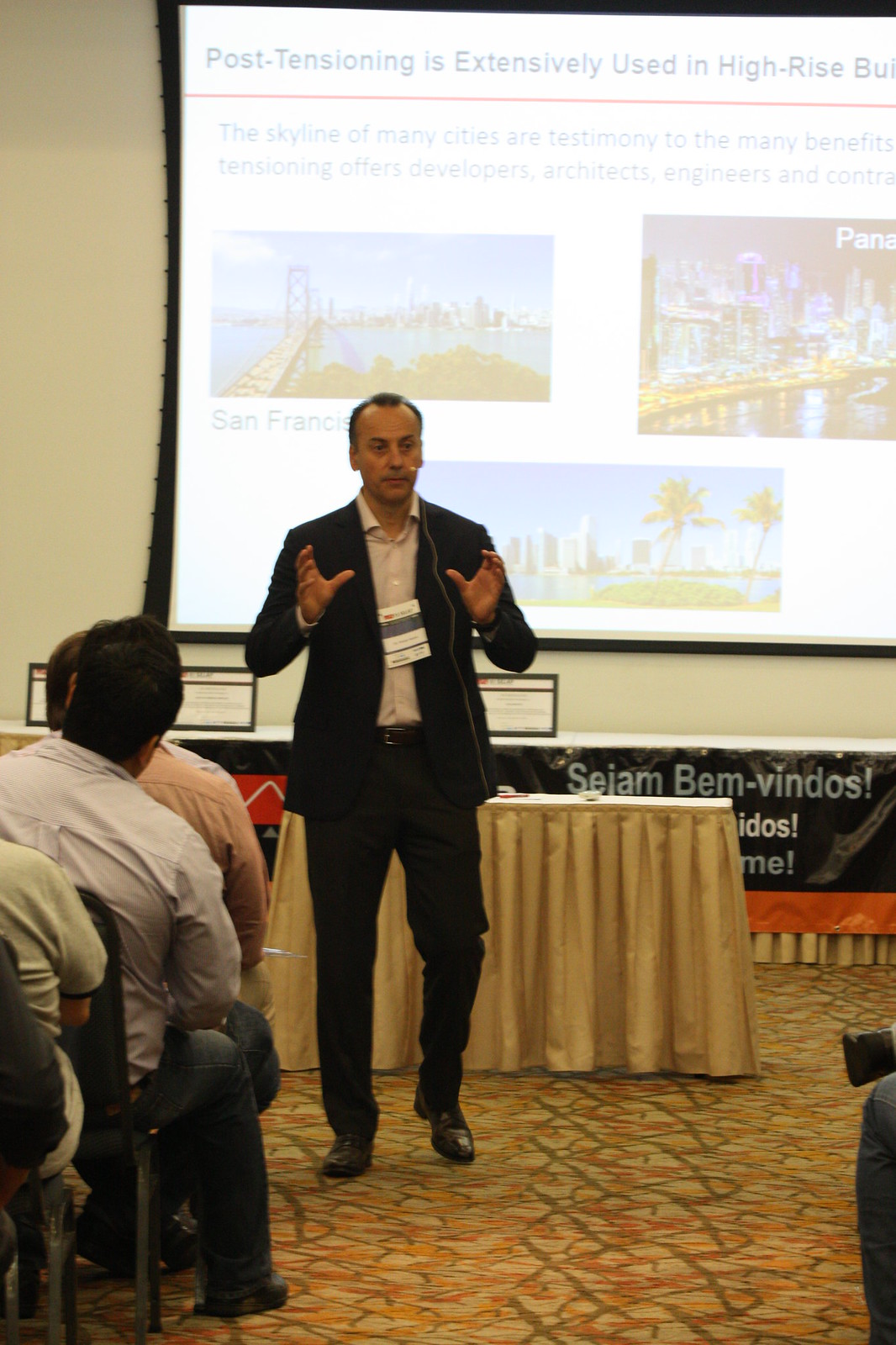A middle-aged Caucasian man, likely in his 50s, is seen speaking passionately at a conference or event, adorned with a black suit and a beige-gray shirt, but no tie. He sports a headset and a name badge around his neck, indicative of his role as the primary speaker. Positioned centrally in the image, he commands the attention of an audience seated on both sides, clearly engaged with his presentation. Behind him, a large white projector screen prominently displays the heading: "Post-tensioning is extensively used in high-rise buildings," along with partial text highlighting benefits to developers, architects, engineers, and contractors. The screen also features images of high-rise buildings, including prominent cityscapes from San Francisco and Panama. The setting appears to be a conference or meeting room, possibly in a hotel or convention center, with a tan tablecloth-draped table and a backdrop of beige pipe and drape that matches the patterned carpet consisting of beige, orange, and dark brown hues.